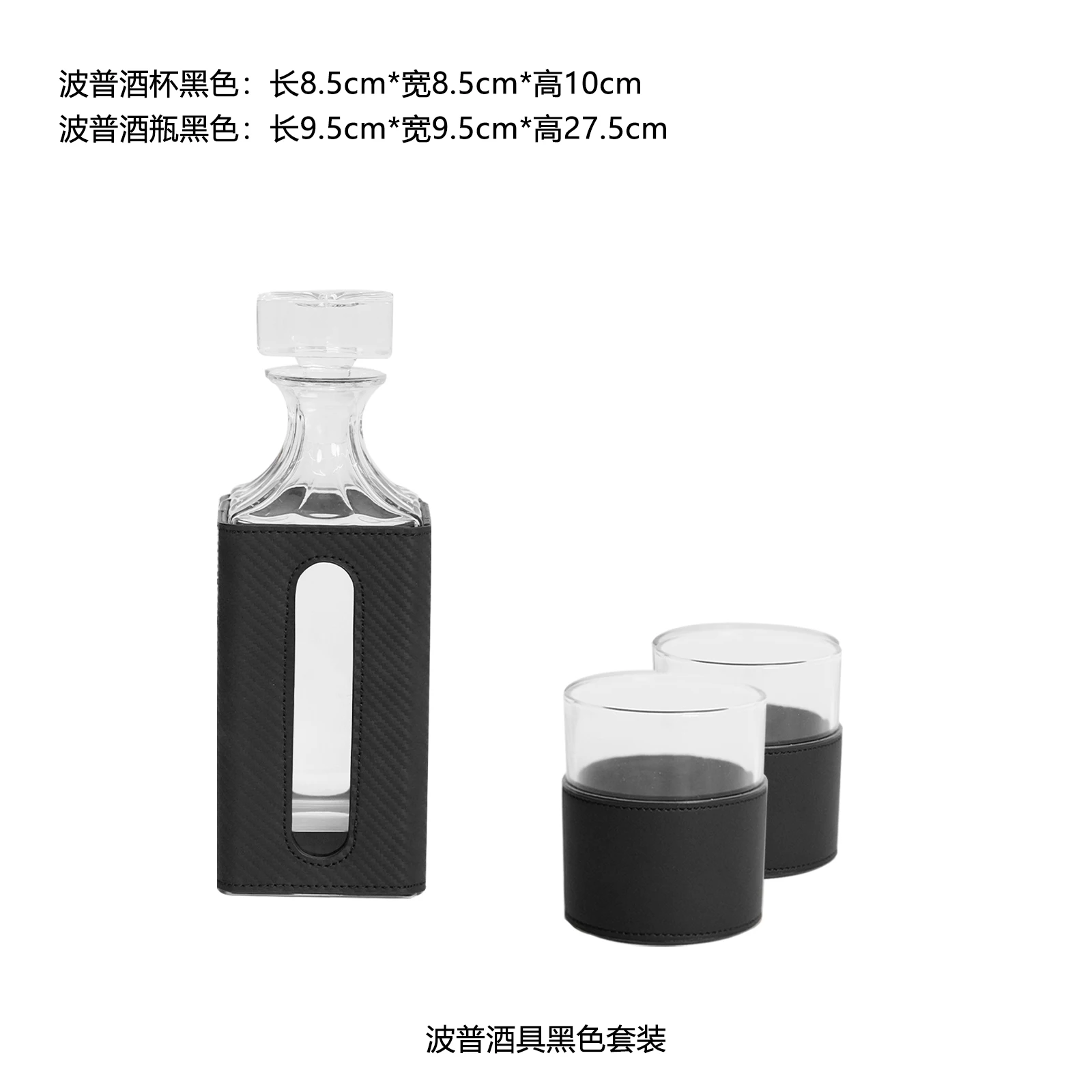The image showcases a sleek, modern liquid decanter and two matching glasses set against a pristine, featureless white background. The central focus is a tall, rectangular-bodied decanter with a flat base and sides, encased in a ribbed dark gray rubber casing with a vertical slit that reveals the liquid inside. The neck of the decanter is crafted from sculpted cut glass and is topped with a rectangular glass stopper. Accompanying the decanter, positioned to its right, are two short, cylindrical glasses. These glasses feature a smooth, dark blue plastic or rubber casing covering roughly the lower two-thirds of their structure, providing a sophisticated and stylish appearance. The top and bottom sections of the image are overlaid with East Asian text, likely Korean, along with numerical details indicating the dimensions of the items: 8.5 cm, 10 cm, 9.5 cm, and 27.5 cm. This image appears to be an advertisement highlighting the design and measurements of the decanter and glass set.